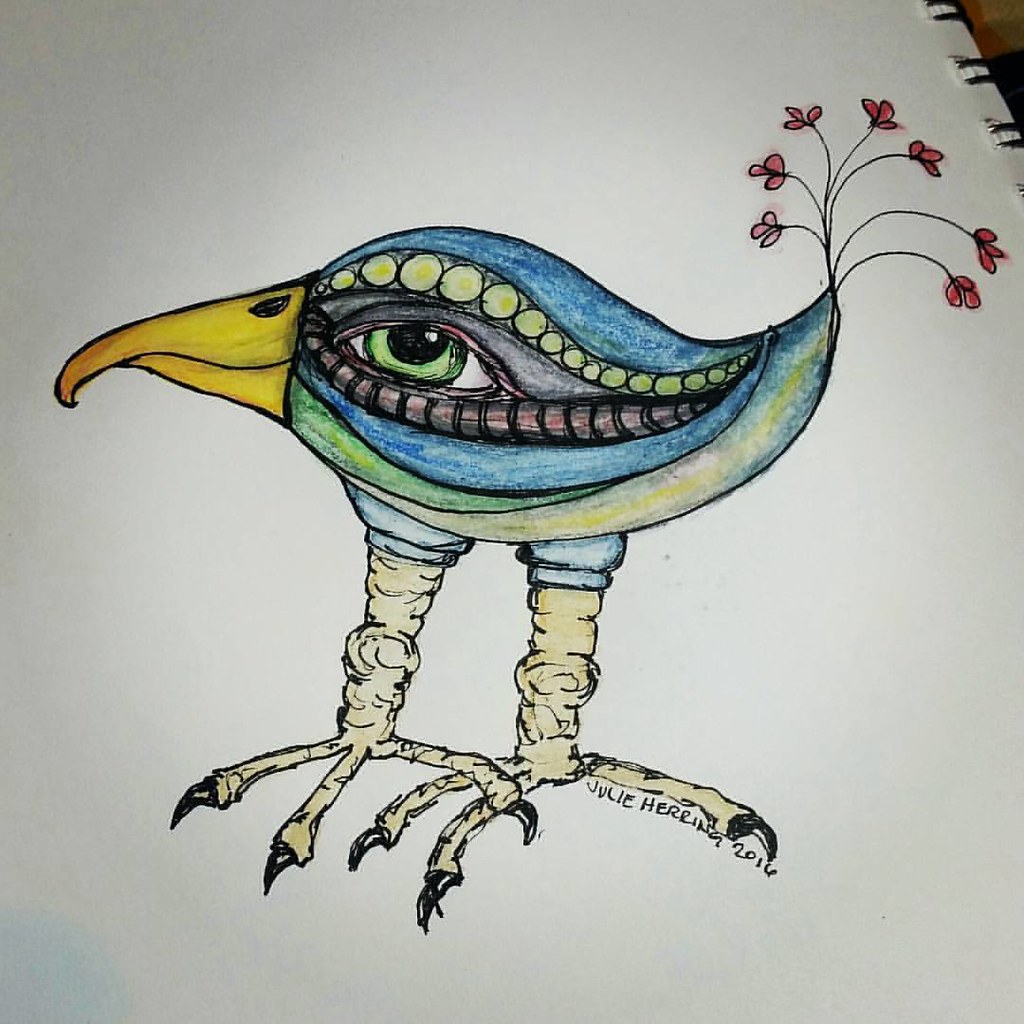This is an unusual drawing executed on a notebook page. The artwork features a peacock with unconventional characteristics. Instead of a separate head, the peacock's head is integrated into its body, with the tail end artistically rendered to resemble a yellow beak. The center of the body contains a striking green eye. Traditional peacock colors are prominent throughout the body, showcasing vibrant blues, greens, and yellows. Emerging from where the head would typically be are seven small, red flowers. The legs are depicted with typical avian features, including three large claws each. Below the claws, there is a signature that appears to read "Julie Herring 2016," presumably identifying the artist.